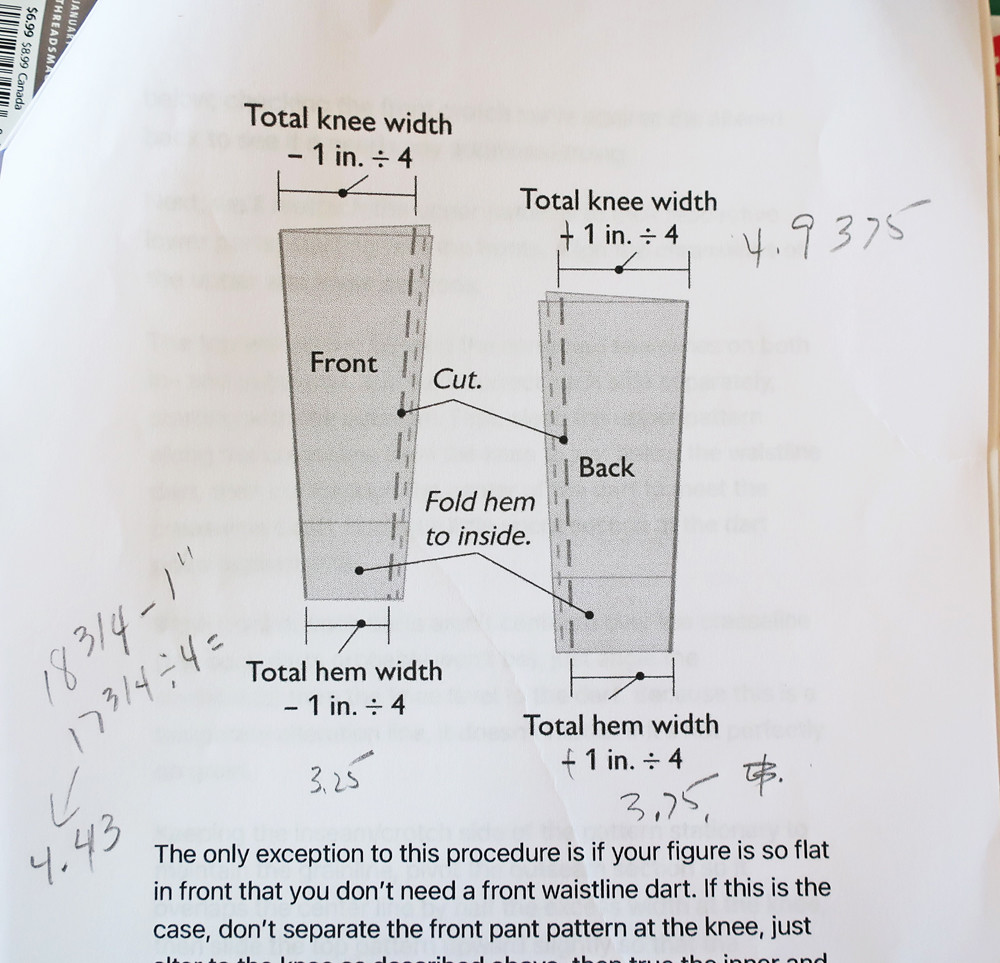This photograph depicts a detailed page from a sewing guide, focused on pants construction. The white page features black diagrams and handwritten notes. Two main diagrams illustrate folded paper patterns labeled "front" and "back." The labels "TOTAL HEMWIDTH" and "TOTAL KNEEWIDTH" are positioned around the images, indicating critical measurement points. Detailed instructions include a note stating, "The only exception to this procedure is if your figure is so flat in front that you don't need a front waistline dart. If this is the case, don't separate the front pant pattern at the knee." Handwritten numbers and pencil calculations are scattered throughout the page, refining measurements such as a total hem width of 3.25 inches. The top left corner of the paper is visibly folded, complementing other calculations noted on both sides for precise tailoring.